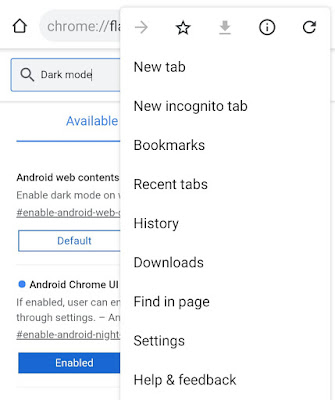This screenshot captures a smartphone display showcasing a website navigated through the Chrome browser. The majority of the screen is dominated by a white background filled with black text, detailing various navigation options within the website. At the very top, a row of icons enhances the navigation experience: a left-pointing arrow for going back, a star for bookmarking, a downward arrow for downloads, an icon for refreshing the page, and an information symbol. Beneath these icons, several navigation choices are listed, including opening a new tab, accessing bookmarks, viewing recent tabs, and checking browsing history. In the backdrop, the design and layout unmistakably reveal the familiar interface of a Chrome browser, further confirming the context of the page.